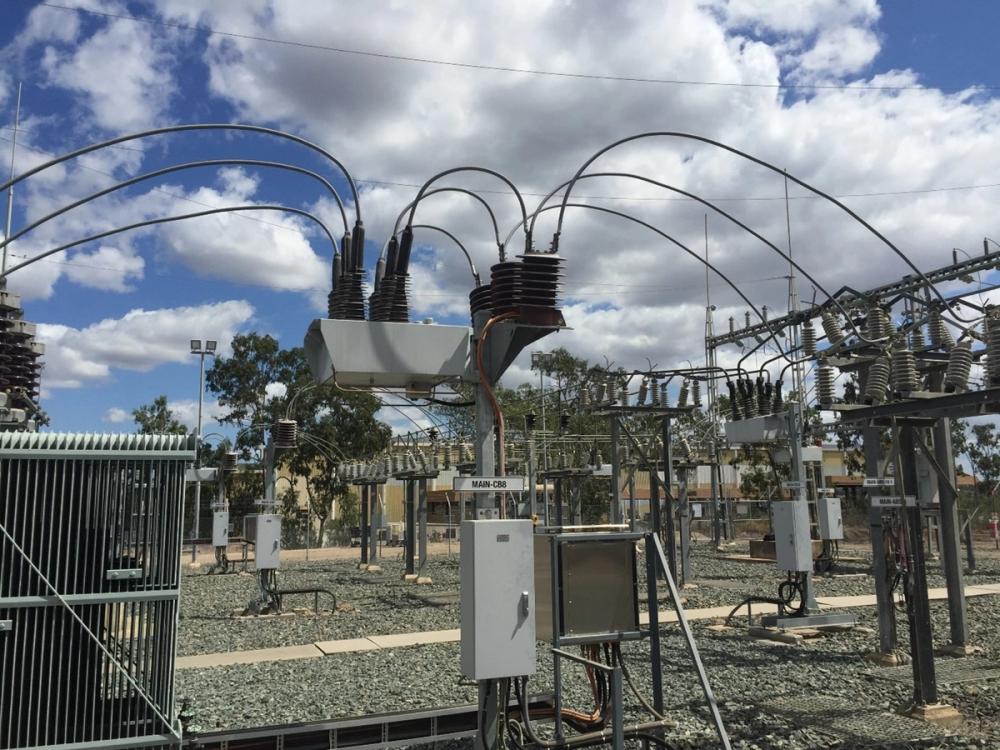This detailed photo captures a power relay station or electric station, characterized by an outdoor setup that includes numerous metal structures and varying types of electrical equipment. The ground is covered with gravel, and there is a narrow sidewalk running through the center, presumably for service workers. Prominent in the image are several transformers, electrical and silver boxes, and ceramic insulators. Metal beams equipped with coils and crossbars are also present, along with large cables that arch and connect various devices.

Notably, the image features a sign reading "MAIN C88," marking one of the transformers, and indicating that each transformer section is labeled. Additionally, there are antennas and what appears to be a large overhead light, likely for nighttime illumination. The fenced-in area is undoubtedly a high-voltage zone, requiring certification and proper safety gear for anyone entering. In the background, trees can be seen under a partly cloudy sky with fluffy white clouds. The presence of these elements suggests it's part of a city's electrical distribution infrastructure.